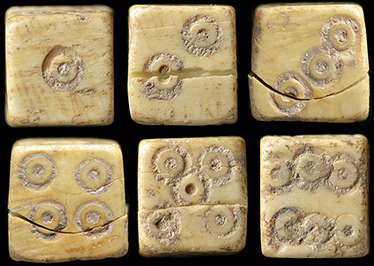The image features a set of six ancient, worn dice or stone artifacts, each displaying the six different faces from one to six, represented by carved circular indentations. The dice are made of a material that appears to be aged ivory, stone, or pottery, with a pale yellowish-beige color and darker, dirt-like marks and streaks suggesting significant wear and historical usage. The circles portraying the numbers are somewhat irregular and not perfectly aligned, further indicating their ancient craftsmanship. Some dice also show deep cut marks and cracks, enhancing their antiquated appearance. The overall arrangement in the image displays all facets of the dice, possibly showing each side of a single die or multiple dice, giving a comprehensive view of these relics from an ancient counting or gaming system.